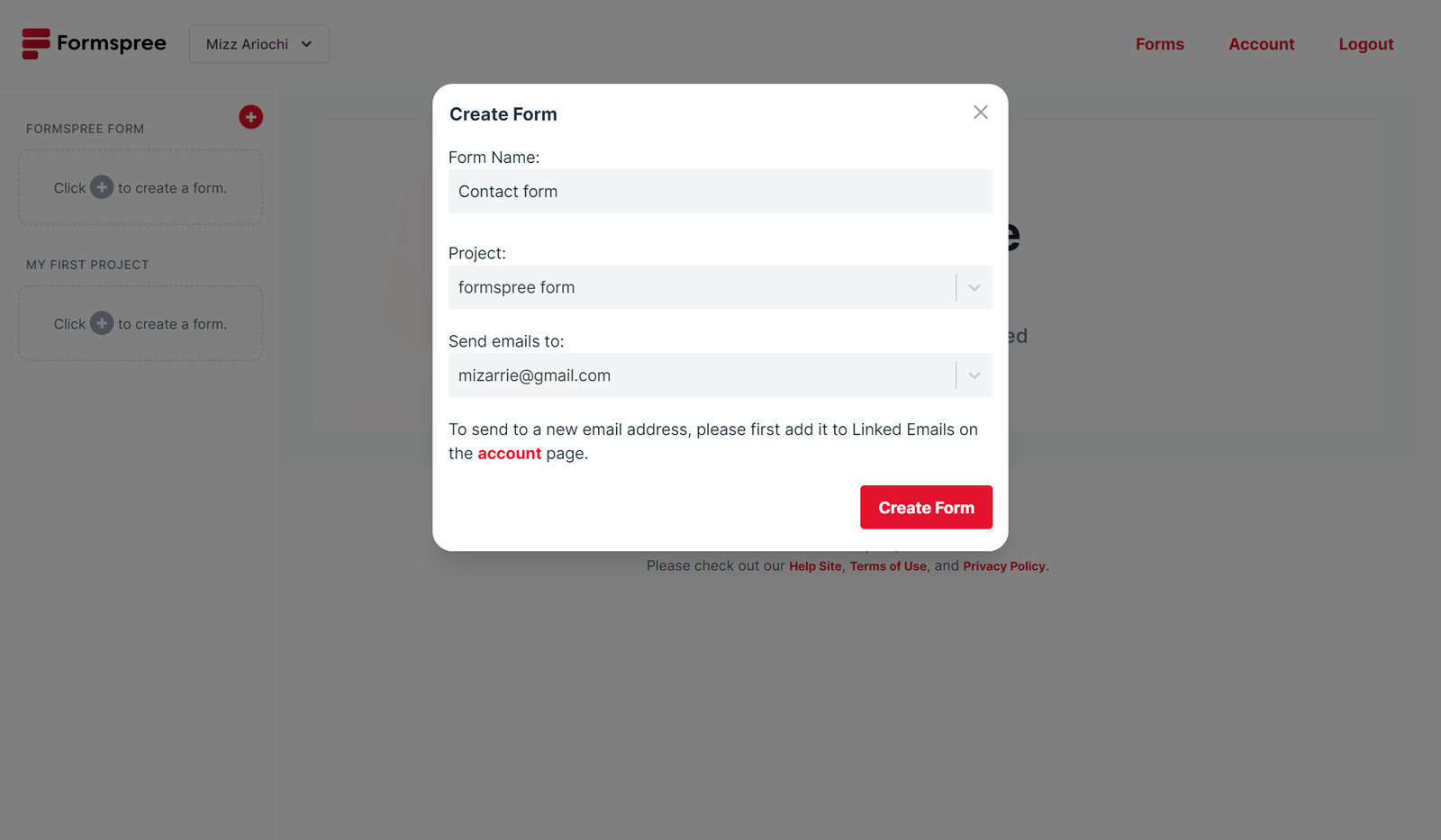In the screenshot, we are navigating the Formspree website where a new form is being created. The interface shows a dialogue bubble with options to input the 'Form Name' and 'Project Name,' as well as specify the email address where form submissions will be sent. Currently, these fields remain unfilled. Below these inputs, there is a prominent red "Create Form" button. The interface also features a red "Account" button, a red "Logout" button, and a red "Forms" button, indicating other available actions in the navigation bar. The overall layout is clean and user-friendly, although the specific purpose of the form being created is unspecified from the screenshot.